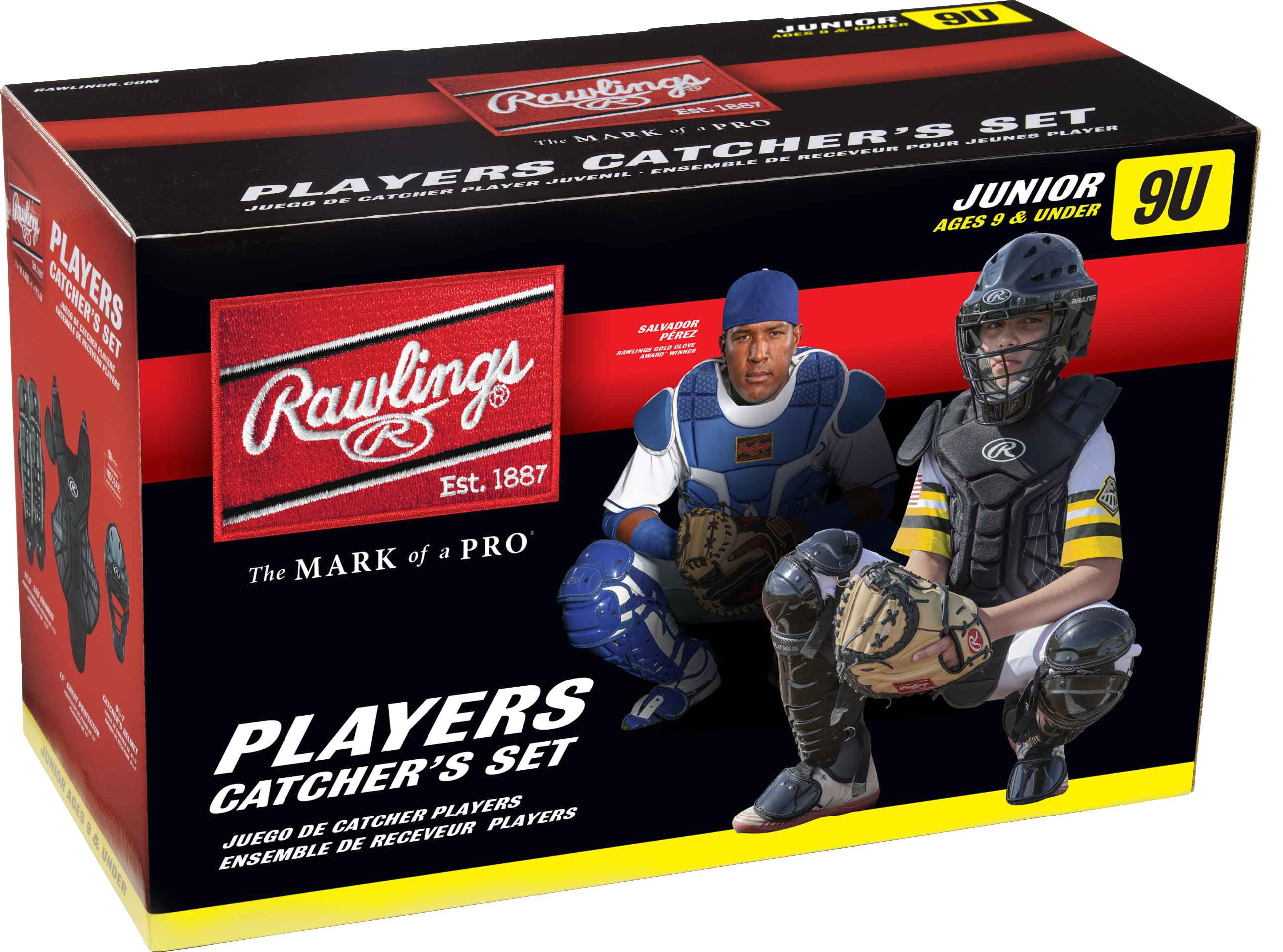The image depicts the front of a red and black rectangular box for a Rawlings junior catcher's set, designed for players aged 9 and under. The box features the Rawlings logo in white, with "EST 1887," "DMARC LB Pro," and "The Mark of a Pro" below it. The product description includes "Players Catcher Set" and its Spanish translation, "Juego de Catcher Players," in white letters. The bottom of the box is bordered by a yellow stripe. The front of the box shows two images: one of a professional catcher, Salvador Perez, and another of a young player in the full catcher's gear—black helmet, chest guard, and leg protectors—crouching in a ready position. The words "Junior" and "Ages 9 and under" are prominently displayed above the kid's image against a gold background with "9U" in black lettering.